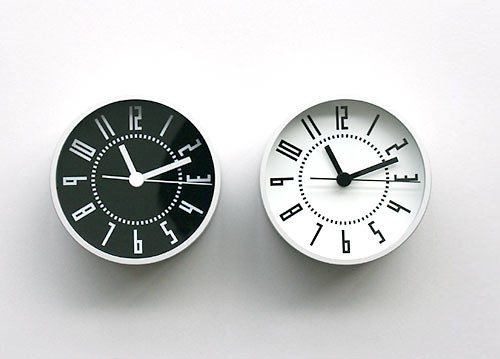In this image, two clocks are positioned side by side, viewed from above, showcasing their front faces. On the left is a black clock with a white outer circle, white hands, and white numerals arranged in a traditional 12-hour format. The hour hand indicates 11, the minute hand is situated between 2 and 3, and the second hand hovers just past the 3 o'clock mark. To the right, a white clock displays black hands and black numerals, mirroring the same time: the hour hand at 11, the minute hand between 2 and 3, and the second hand just past the 3. Both clocks rest against a gray background that gradates from darker shades at the bottom to lighter shades at the top.